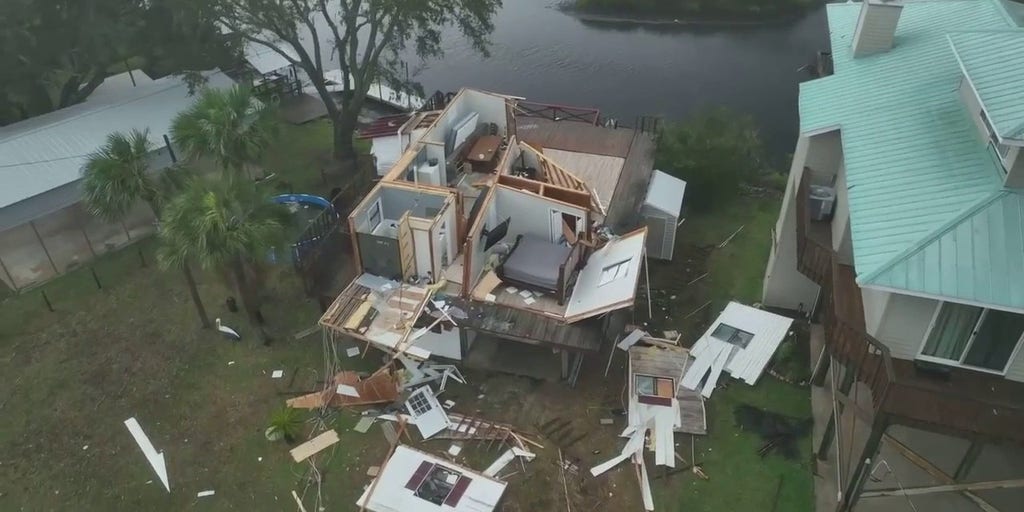In this detailed aerial photograph, likely captured by a drone during the daytime, we see a vivid aftermath of a severe storm. Central to the image is a house that has been catastrophically wrecked, with its roof completely missing, revealing the disarray inside. Furniture and debris are strewn across the rooms and the surrounding yard, with some parts blown over to a neighboring property. This neighboring house, positioned to the right, remains mostly intact with a mint green roof and an undamaged deck, standing in stark contrast to the devastated home. The flooded streets and a body of water, possibly a lake or river, visible in the background suggest the storm brought significant flooding. Surrounding the scene are palm trees and other greenery, with one tree on the left harboring a white bird on the ground beside it. A blue item, resembling a kid's pool, is also noticeable near the base of the trees. The diverse palette in the image includes teal, brown, white, black, dark green, blue, and beige, highlighting the chaos and natural vibrancy of the post-storm landscape.